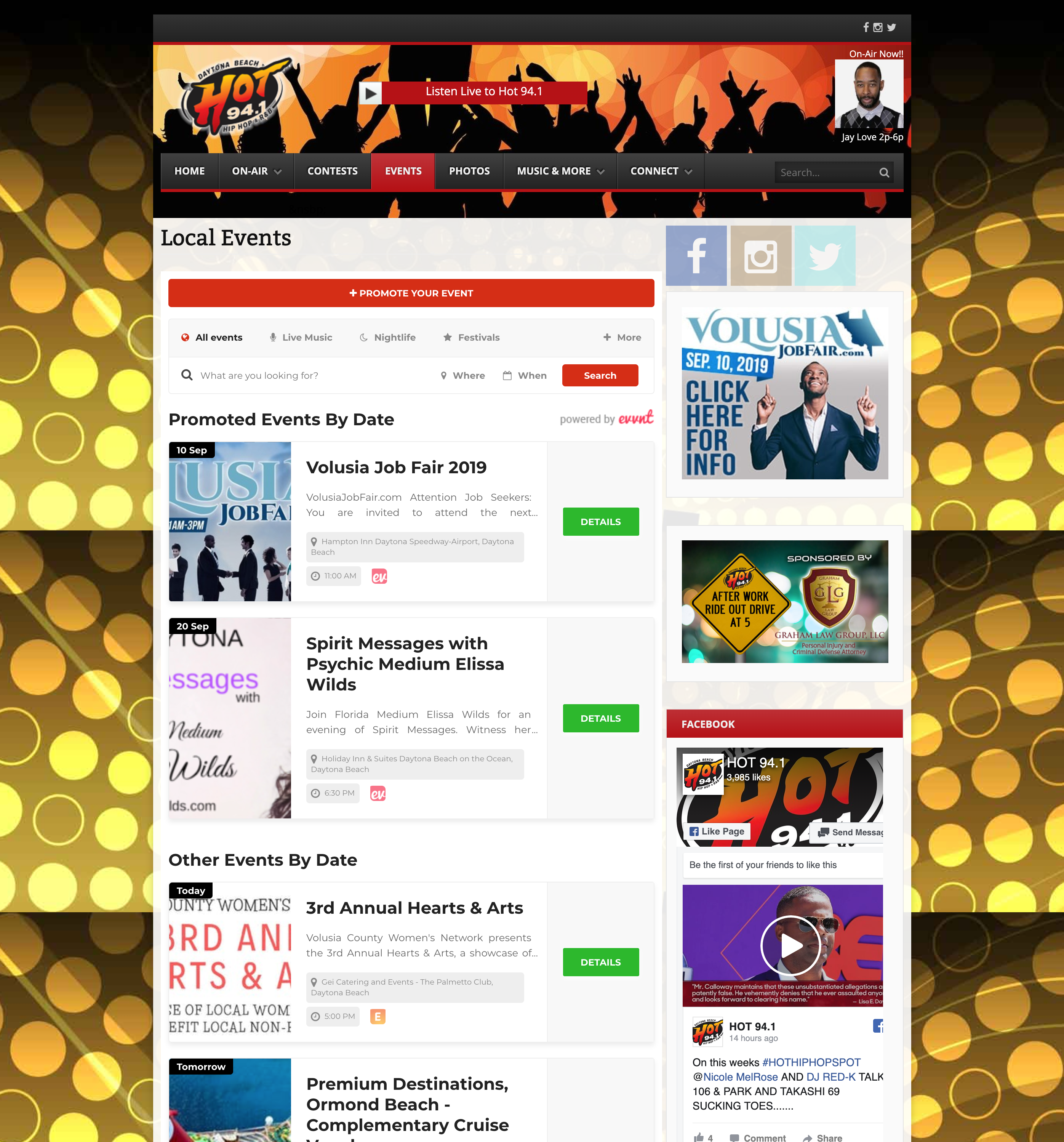A radio station broadcast from Daytona Beach-based HOT 94.1, dedicated to Hip Hop and R&B genres. The station features various categories such as On Air segments, Contests, Events, Photos, Music, and more. Currently on air is JLOVE, hosting from 2 PM to 6 PM. The station also connects listeners with local events, offering options like Live Music, Nightlife, and Festivals, as well as promoted events by dates, including the Volusia Job Fair 2019, Spirit Messages with Psychic Medium Elisa Wilds, and Dead or Not Hats and Hats. The station prides itself on being a premium destination among beachgoers, offering complimentary coverage of this week's hottest hip hop spots.